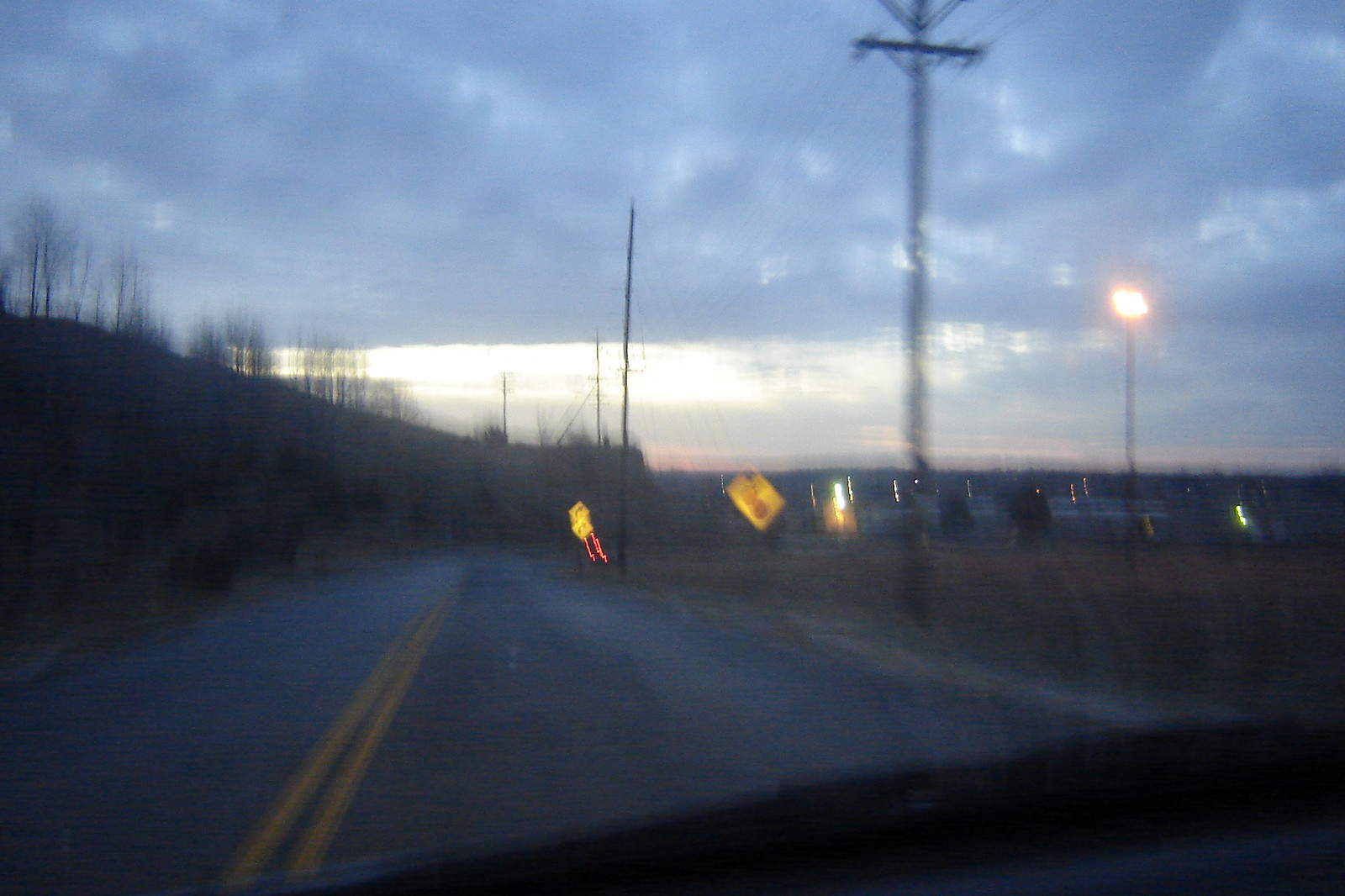This Polaroid captures a rural road scene through a car windshield at dusk, with the sky transitioning to nighttime. The windshield itself is clean, but the scene outside is blurry, creating a double-vision effect. The road stretches out ahead with a double yellow line, having one lane in each direction. There are a few streetlights, along with normal street signs and some yellow traffic signs, including one with a red dot and another with red lights underneath it. The sides of the road are flanked by grass and a slight hill on the left. Electrical poles with wires extend along the road. Thick, dark clouds dominate the top of the sky, partially covering the bright orange sun, which reflects off the clouds. In the distance, the faint lights of a town can be seen along with some buildings. An orange light is visible atop a pole in a nearby field. The image suggests it's close to 8 PM.